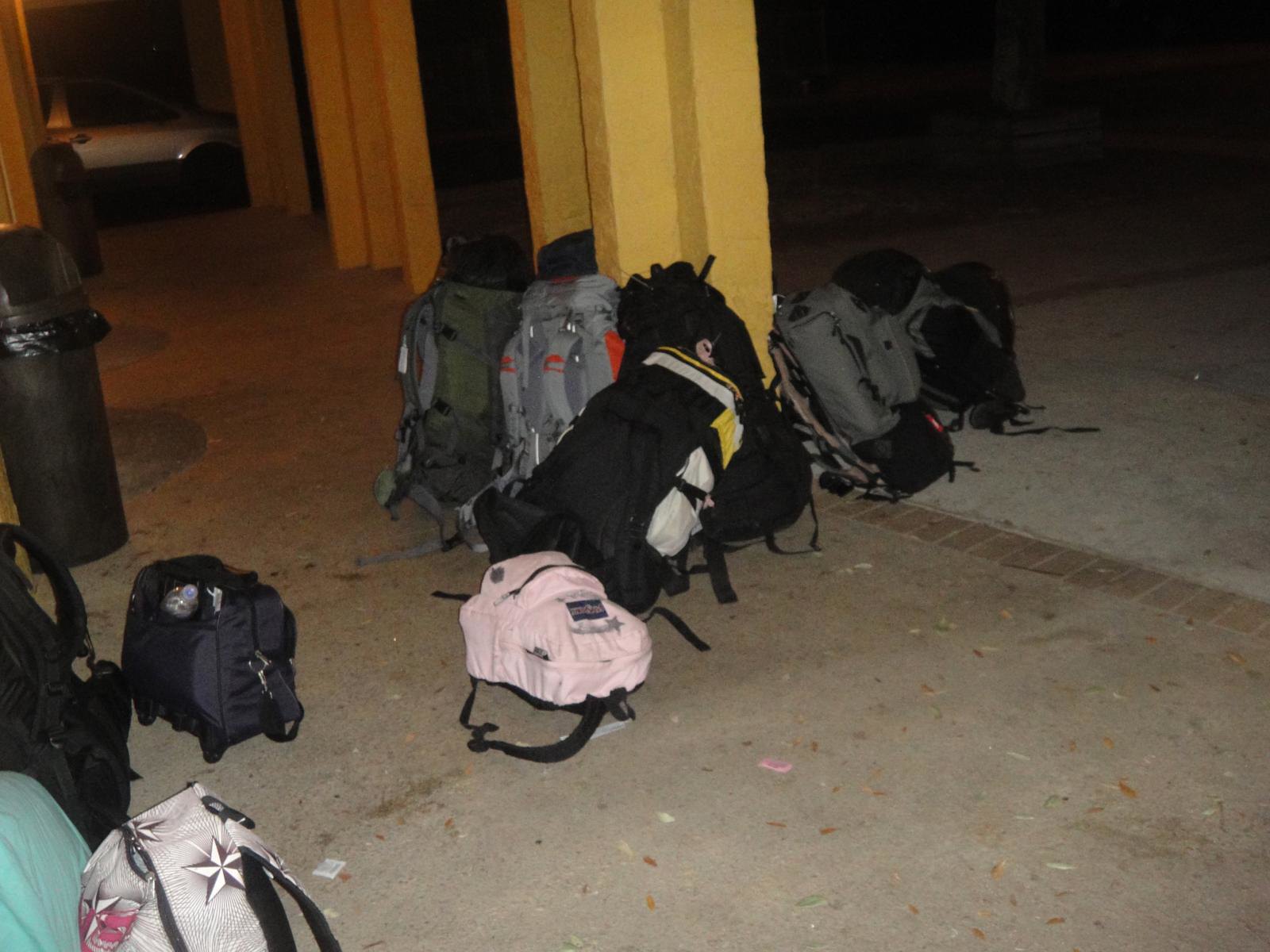In this rectangular landscape image, a collection of approximately 11 backpacks is arranged on a concrete floor in what appears to be an empty corridor or parking garage. The focal point of the scene includes large yellow structural support beams, around which the bags are clustered. The backpacks are primarily of the backpacker variety, characterized by their long, rectangular shapes and colors such as green, gray, and black. Noteworthy among them is one normal-sized school backpack lying flat with a recognizable Jansport logo. Flanking the left side is a black-brown trash can with a black garbage bag inside. In the background, a white car can be seen through a passageway, enhancing the sense of emptiness in the setting. The variety in the backpacks is notable: alongside the predominantly green and gray tall backpacks, there are additional bags featuring star patterns, wheels, and diverse colors such as red, teal, pink, and even pink and white. The scene, devoid of people, emphasizes the stillness and abandonment in this concrete and steel environment.